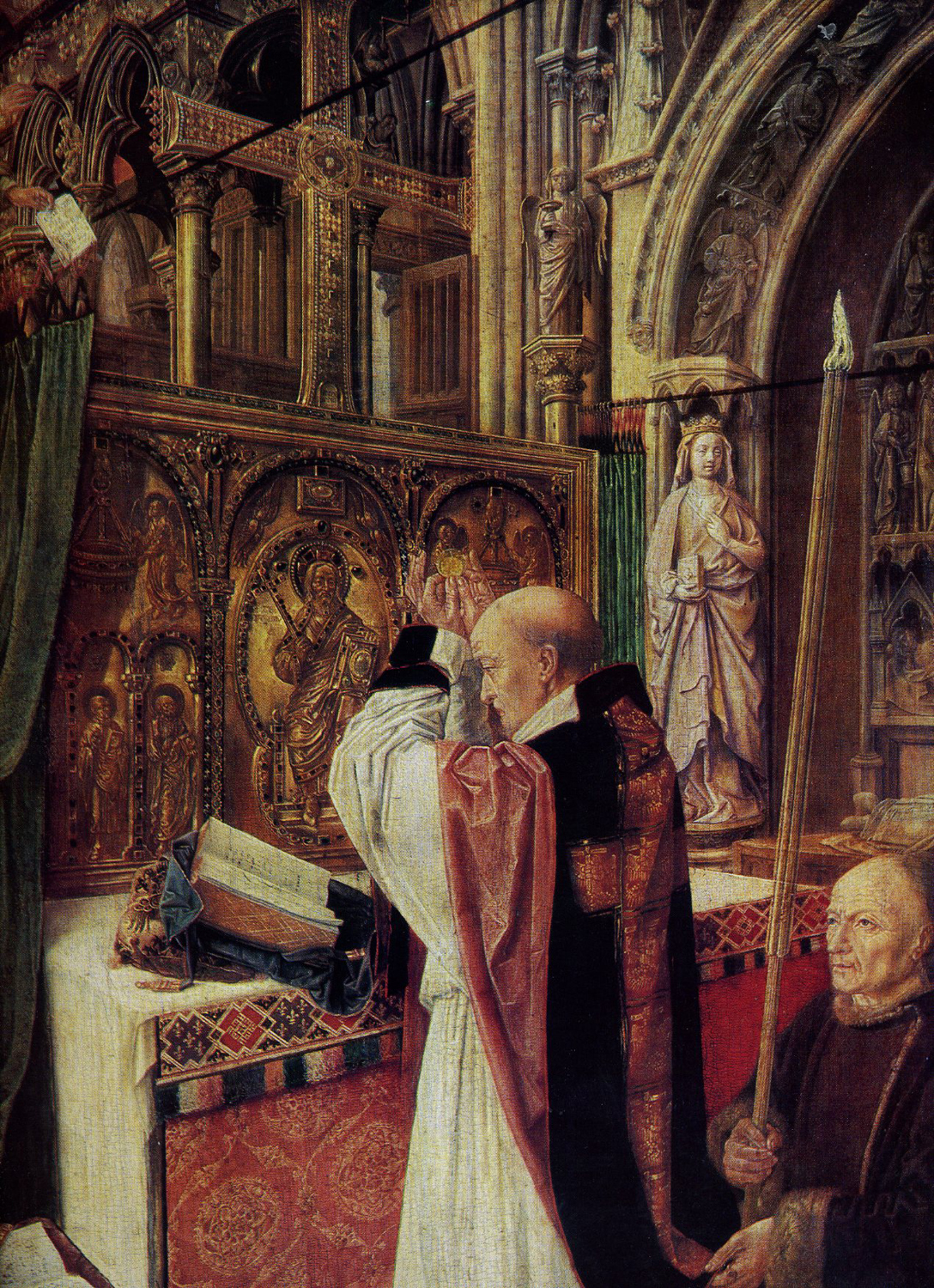The image is a detailed painting from early antiquity, possibly around 800 BC or AD, depicting a religious scene inside a Gothic-style Catholic church. Central to the artwork is a priest, dressed in traditional garb including a burgundy cape and a white gown, standing at the altar. His arms are raised, and he appears to be reading or praying from an open Bible placed on the altar, which is adorned with altar cloths. Religious imagery is abundant throughout the scene, featuring prominent Catholic icons such as a cross and a statue of the Virgin Mary to the right of the priest. In the background, a second man, dressed in black robes, sits or crouches while holding a long pole or scepter-like object that may have a fire at its tip. This solemn assistant, with a neutral expression, seems to be part of the religious ceremony. Ornate statues, including angels and other religious figures, embellish the church's architecture, adding to the painting’s intricate and reverent atmosphere.